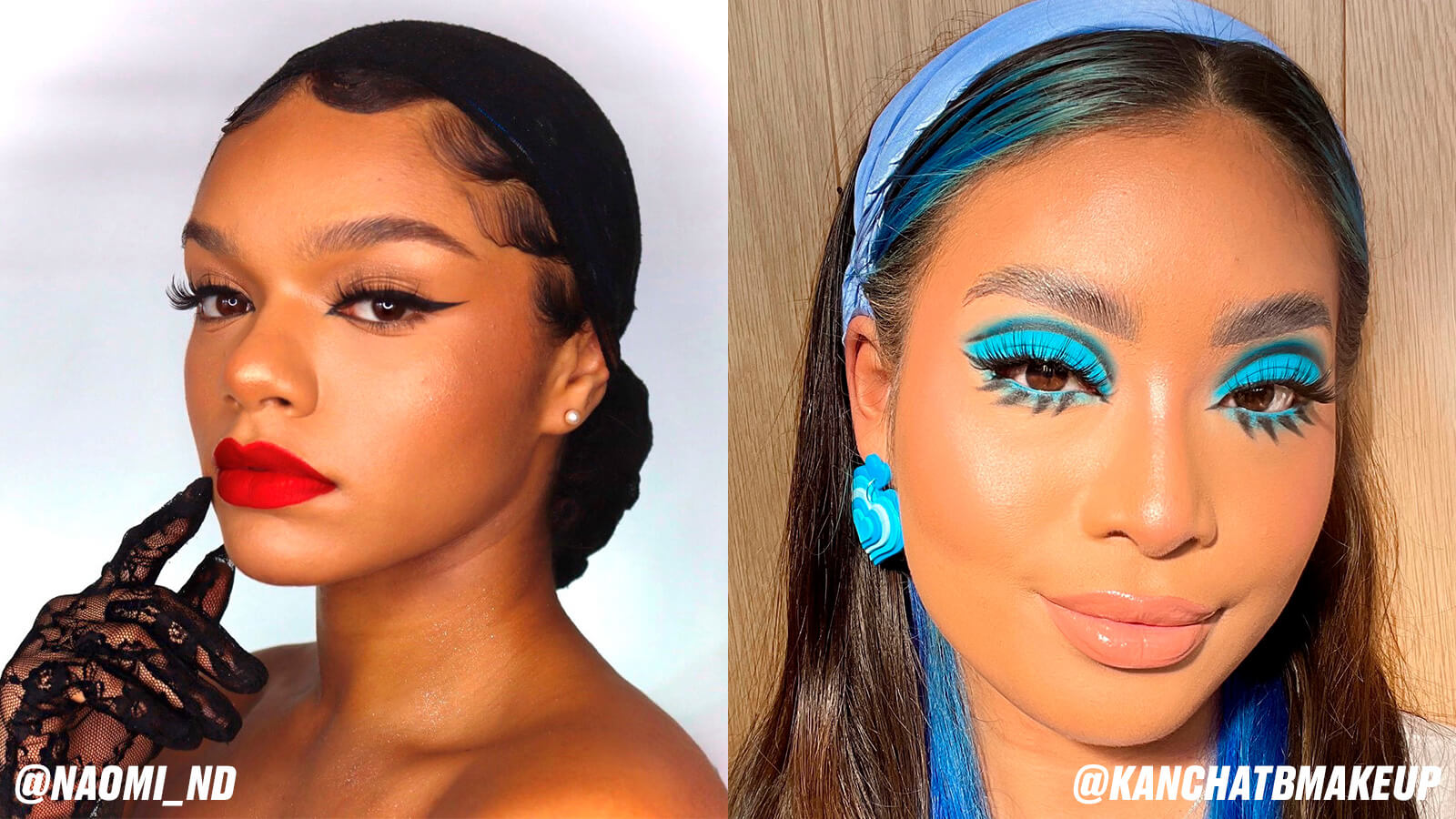This image is a horizontal rectangular, side-by-side composition featuring two darker-skinned women, each heavily adorned with makeup. Both women have smooth skin and are looking directly at the camera.

On the left side, the woman tagged as @Naomi_ND is a black woman with her black hair swept back, mostly resting on the back of her neck. She is wearing a black cap and appears to have her hair pulled back possibly with a head wrap. Her makeup includes prominent cat's eye eyeliner, false eyelashes, and very dark red lipstick. Her eyebrows are thick and drawn in. She is adorned with pearl earrings and is wearing dark gloves or stocking-style gloves on both hands, with two gloved fingers touching her face. You can only see up to her clavicle and shoulders, without any visible clothing.

On the right side, the woman tagged as @CanChatBeMakeup has long dark hair with striking blue highlights and a tiny part. She is wearing a blue headband and blue, heart-shaped earrings with white accents. Her makeup is consistent with a blue theme: heavy blue eyeshadow, blue eyeliner, and likely false lashes. Her perfectly thick eyebrows stand out, along with a natural skin tone accentuated by glossed pink lipstick. The lower corners of the image contain the respective tags for each woman, affirming their identities and the distinct makeup details.